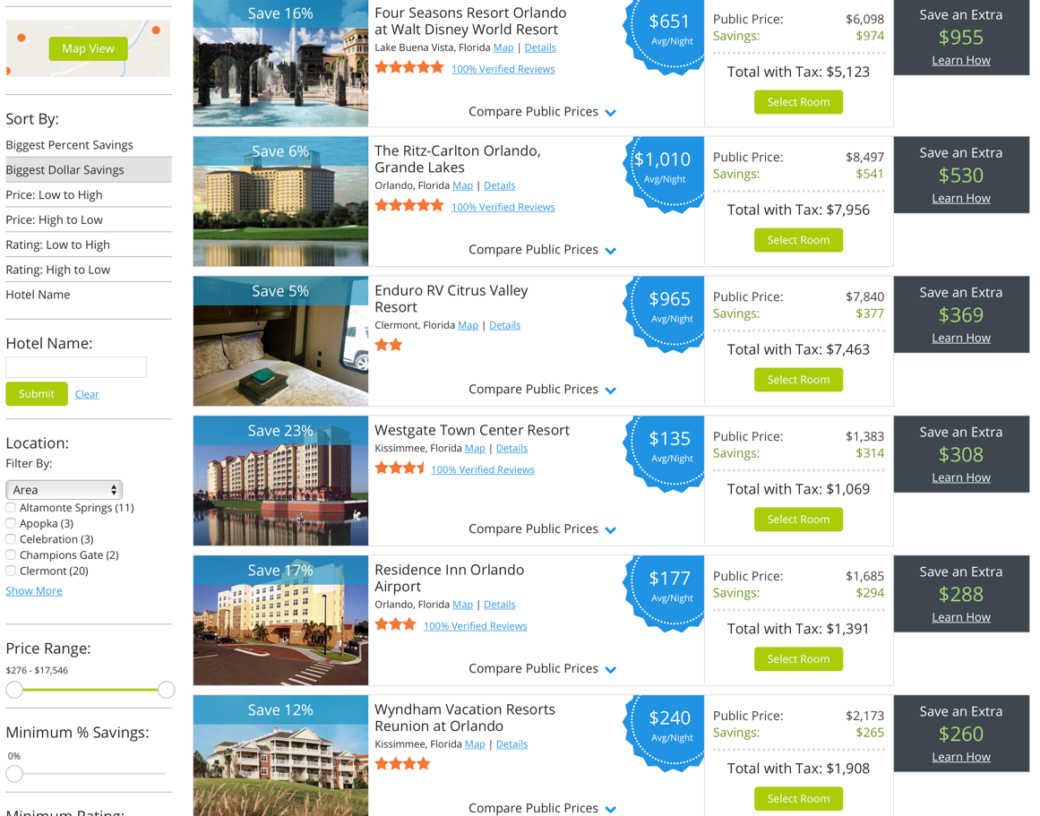A screenshot of a resort booking website is displayed, showcasing various options and filters for users seeking accommodations. On the left side of the screenshot, an extensive filter panel is presented:

- **Map View:** Allows users to visualize the resort's location on a map.
- **Sort By Selection:** Various sorting options are available, with the current selection being "Biggest Dollar Savings."
- **Hotel Name:** Includes fields for entering and filtering by the hotel name along with 'Submit' and 'Clear' buttons.
- **Location:** Filter by location with the current filter set to 'Area'. Additional filtering options are available via a "Show More" button.
- **Price Range:** The selected range is $276 to $17,546.
- **Minimum Percent Savings:** Currently set to 0%.
- **Minimum Rating:** The filter is partially visible, cutting off the selected value.

In the main area, six resorts are featured. Each listing provides comprehensive details:

- **Title and Location:** Names and geographic locations of the resorts.
- **Customer Reviews:** Ratings on a 5-star scale.
- **Average Price per Night:** Estimated nightly rates.
- **Coupons and Savings:** Opportunities for additional discounts and public price comparisons.
- **Room Selection:** An option to book a room at each resort, marked by a prominent green button.

This organized layout aids users in making informed decisions by offering a wide array of sorting and filtering tools, ensuring a seamless resort selection experience.